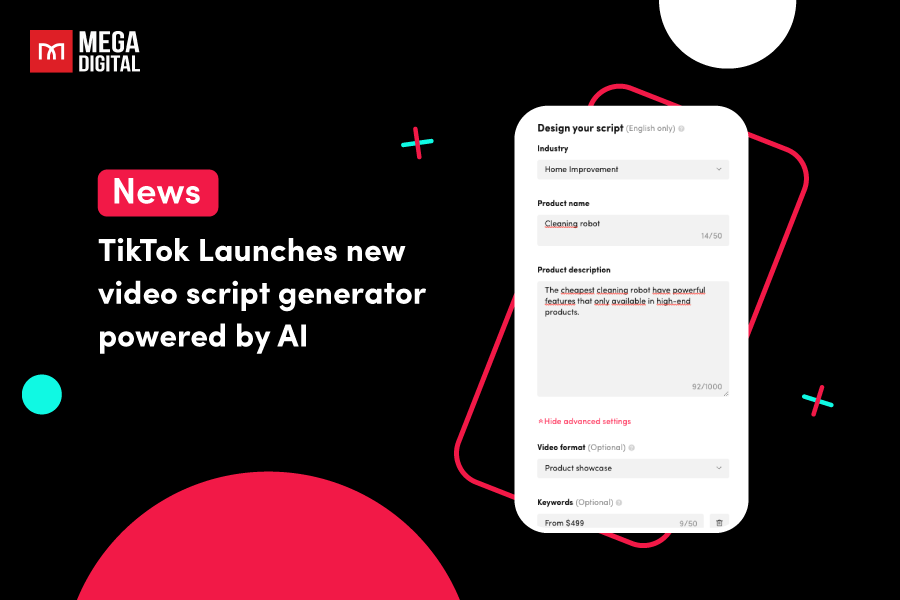The image depicts a promotional advertisement launched by TikTok, featuring their new AI-powered video script generator. Dominating the right half of the page, a sleek, interactive interface is showcased, illustrating how users can design their scripts. The top left corner prominently displays the Mega Digital logo with the phrase "Mega Digital" written alongside. Just beneath this, a bold headline declares, "News: TikTok launches new video script generator powered by AI." Scattered throughout the advertisement are TikTok’s iconic colors, reinforcing the brand’s identity. The minimalist background features two crosses and three circles, maintaining focus on the promotional content. Overall, this advertisement from TikTok aims to highlight the innovative new feature available on their platform.